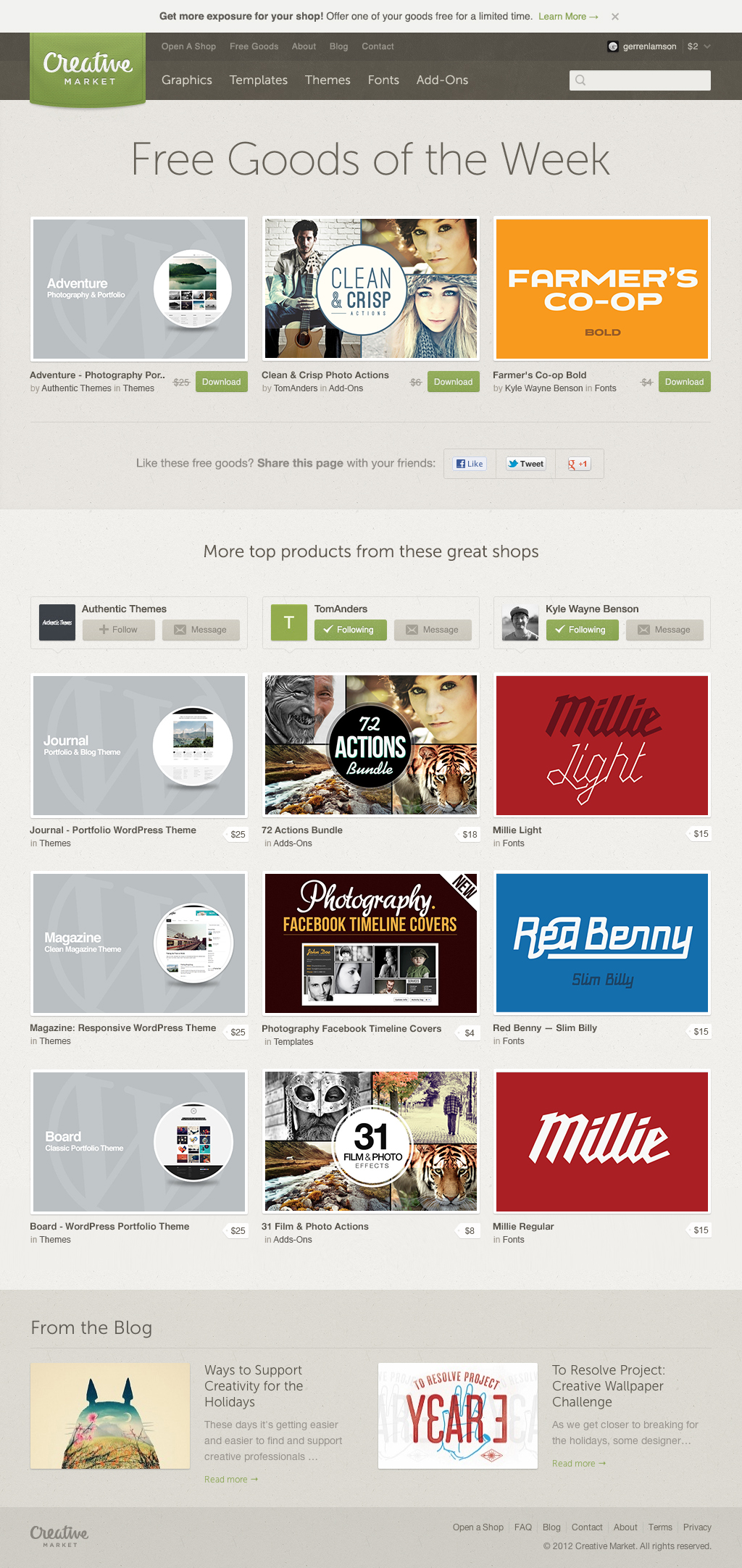The image showcases a gray background and seems to be a screenshot of a website, with a detailed, albeit somewhat cluttered, layout. At the top in black text, it says, "Get more exposure for your shop. Offer one of your goods free for a limited time." Below this is a black banner that features a green area on the left with the logo "Creative Market." 

The banner includes tabs for navigating the site, labeled: "Open a Shop," "About," "Blog," "Contact," "Graphics," "Templates," "Themes," "Fonts," and "Add-ons." Adjacent to these tabs, there is a search bar. 

Beneath the banner, there is a beige section labeled "Free Goods of the Week," which features three images with text descriptions beneath them. Further down, a larger header reads "More top products from these great shops," followed by a grid of nine thumbnails.

The thumbnails are organized into three columns: 
- On the left, against a gray background, the images are labeled "Journal," "Magazine," and "Board."
- In the center, featuring images of people and animals, the items are named "72 Action Bundle," "Photography," "Facebook Timeline Covers," and "31 Film and Photo."
- On the right, three colored boxes (one red, one blue, and another red) display the names "Millie Light," "Red Binnie," and "Millie" in white text.

At the bottom, a tan background area highlights three blog post titles: "Ways to support creativity for the holidays," "To Resolve Project," and "Creative Wallpaper Challenge."